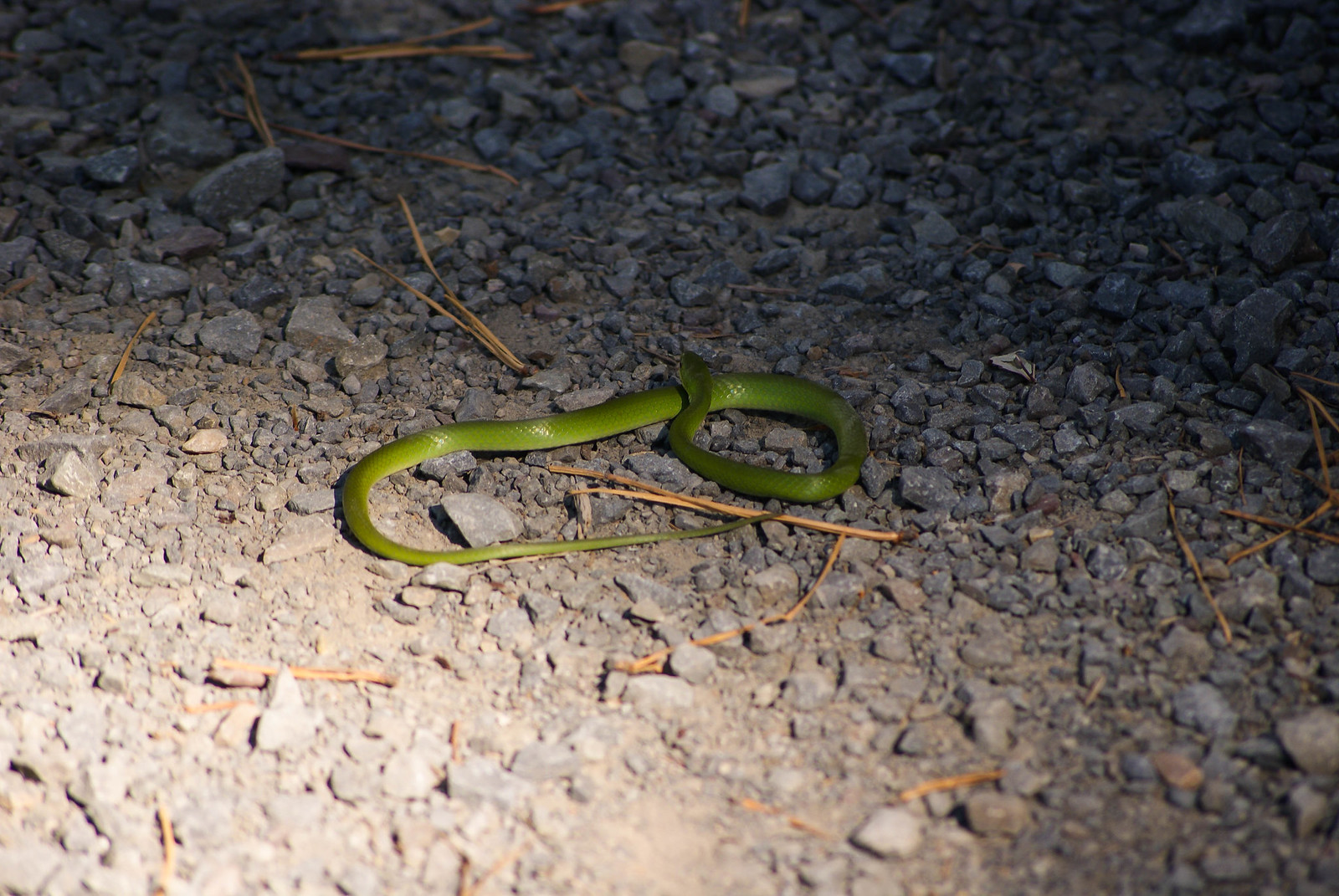This color photograph captures a solitary, vibrant green snake coiling gracefully amidst a rocky, gravelly terrain under the stark illumination of a spotlight or flash, likely taken outdoors at night. The snake, positioned prominently in the mid-ground of the image, displays a beautiful two-tone green hue, its scales glistening in the light. It is loosely coiled, with its head resting on its own back, looking away from the camera. Surrounding the snake are numerous grey stones and a scattering of brown pine needles and twigs, contributing to an intricate backdrop of contrasting textures. In the background, more dark grey stones and an orange branch can be seen, adding to the natural and somewhat serene scene. Despite its setting on a rugged surface, the snake exudes a non-threatening, almost friendly demeanor, accentuated by its harmonious placement within the image.